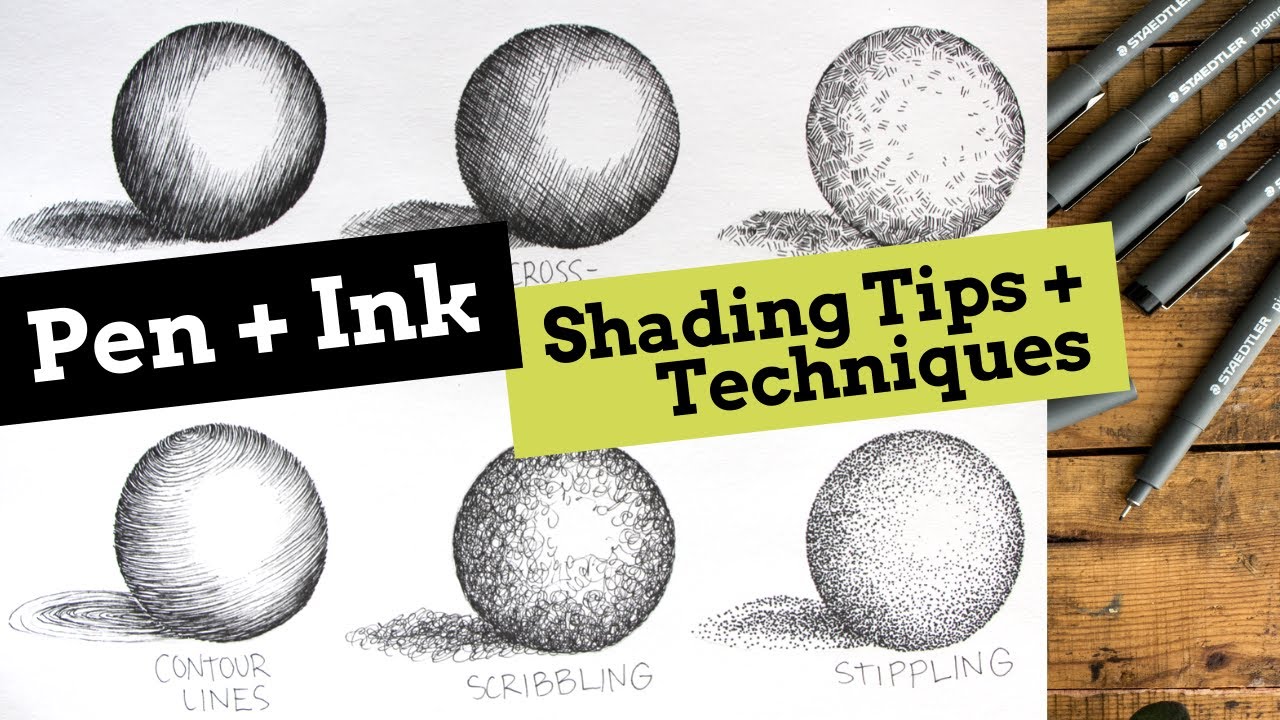The image appears to be the cover of an instruction book on pen and ink shading techniques or possibly an advertisement for the same. The layout is a horizontal rectangle. The majority of the frame, roughly five-sixths, is dedicated to pen and ink drawings of six different spheres, showcasing various shading methods. Each sphere has a unique style of shading: the three at the bottom are labeled "contour lines," "scribbling," and "stippling" in block print. Overlaying the spheres are two banners: a black bar with white text reading "pen + ink" and a green bar with black text reading "shading tips + techniques."

On the right side of the frame, occupying about 20% of the image, is a photograph of five black pens placed on a brown wooden tabletop. The pens, identifiable as Staedtler brand, are arranged in a loose, vertical row. Four of the pens are angled from the left up towards the right, with parts extending out of the image frame. A fifth pen lies below them, pointing from right to left, with its fine tip visible at the bottom.